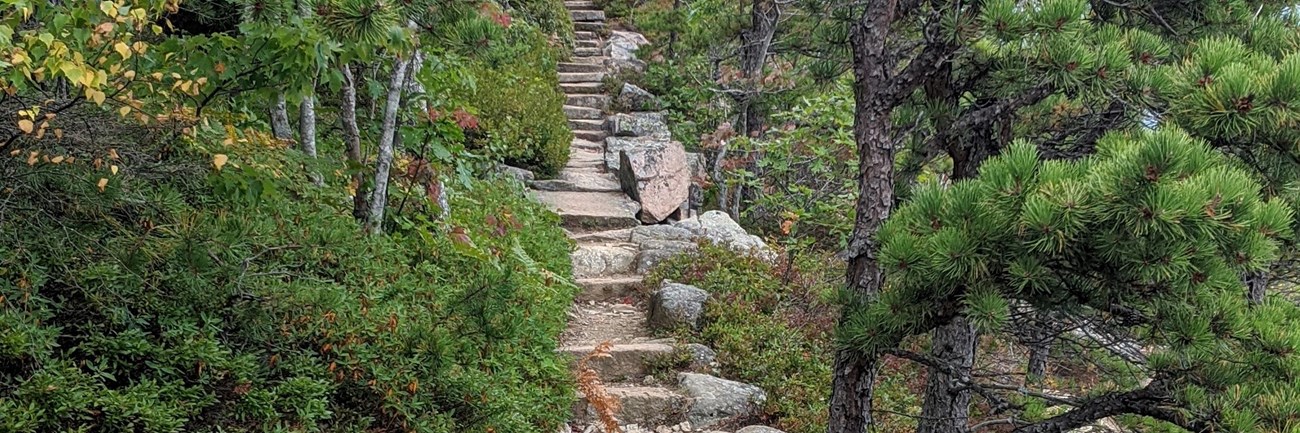The photograph features a scenic stone walkway, composed of large, unevenly placed gray stones forming steps that create a charming path ascending through a picturesque, semi-tailored garden reminiscent of a Japanese landscape. The path begins in the lower middle of the image and extends upwards past the top middle, meandering slightly to the right. Alongside the steps, on the right, several large boulders made of light brownish-gray stone are arranged, serving both an aesthetic and practical purpose to prevent erosion on the gently sloping terrain that descends to the right. 

To the right of the walkway, there are tall, thin trees adorned with bright green needles, creating a vibrant contrast against the stones and enriching the garden's lush greenery. A small patch of green grass and brown dirt ascends towards the top of the walkway, blending seamlessly with the natural elements. On the left side, clusters of lower green bushes and a few white trees add to the landscape's diversity and visual appeal. 

The entire scene is bathed in natural daylight, highlighting the carefully organized plants and the meticulously crafted path, creating a serene and inviting atmosphere in this tranquil outdoor setting.